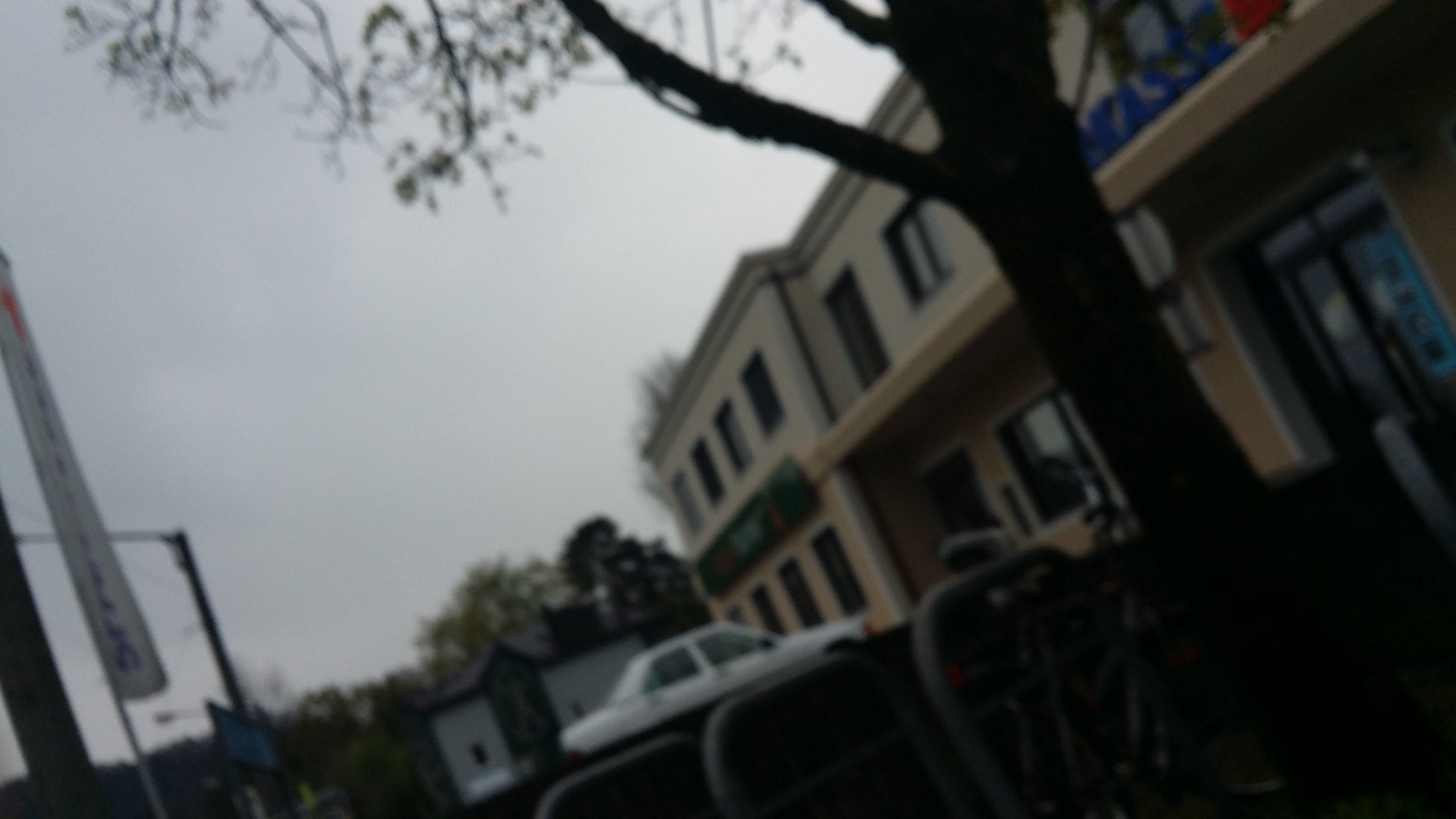This out-of-focus photograph captures an outdoor area adjacent to a retail establishment. Dominating the center of the image is a white sedan parked in front of a tan, two-story building, which houses various retail shops on the ground floor. A leafless tree, suggesting the season is either early spring or late fall, stands in the foreground, partially obscuring what appears to be a set of chairs or a bike rack. The sky on the left side of the image is overcast, casting a gray tone over the scene. Vertical signs are also visible on the left, adding to the commercial ambiance of the setting.